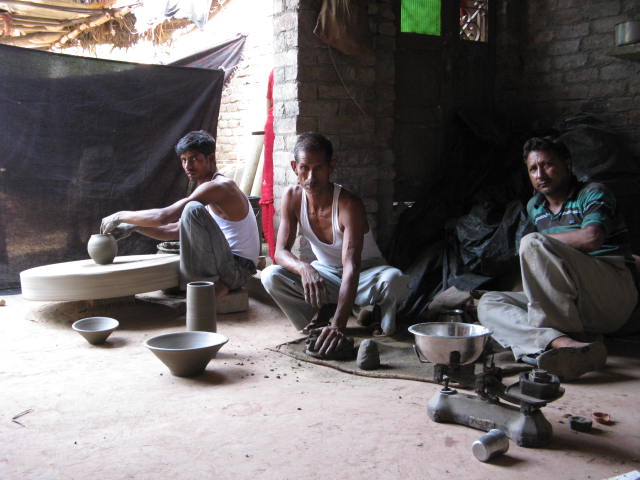In this image, we see three men of likely Indian descent engaging in pottery work outside a dilapidated brick building. The man in the center, wearing a white singlet and beige trousers, has grey, dirty hands as he molds a piece of clay on a spinning pottery wheel. To his left, a man in a similar white singlet and white trousers stares directly at the camera, with muscular arms and a mustache. He appears to be engrossed in mixing clay in a silver metal bowl. On the far right, a tired-looking elderly man reclines, wearing a green and black striped shirt with beige trousers and sandals. He is also involved in the pottery process, perhaps supervising or resting between tasks. Several finished clay pots and bowls are visible on the ground around them, indicating their craft. The scene is set against a backdrop of a partially visible brick building, with black tarps or nets hanging from the walls, creating a sort of barricade and contributing to the dim lighting. The overall environment suggests a humble, possibly impoverished setting, with elements like a grey floor and scattered trash reinforcing the sense of a third-world locale. All three men appear focused on their work, contributing to the rich cultural tapestry of traditional pottery-making.